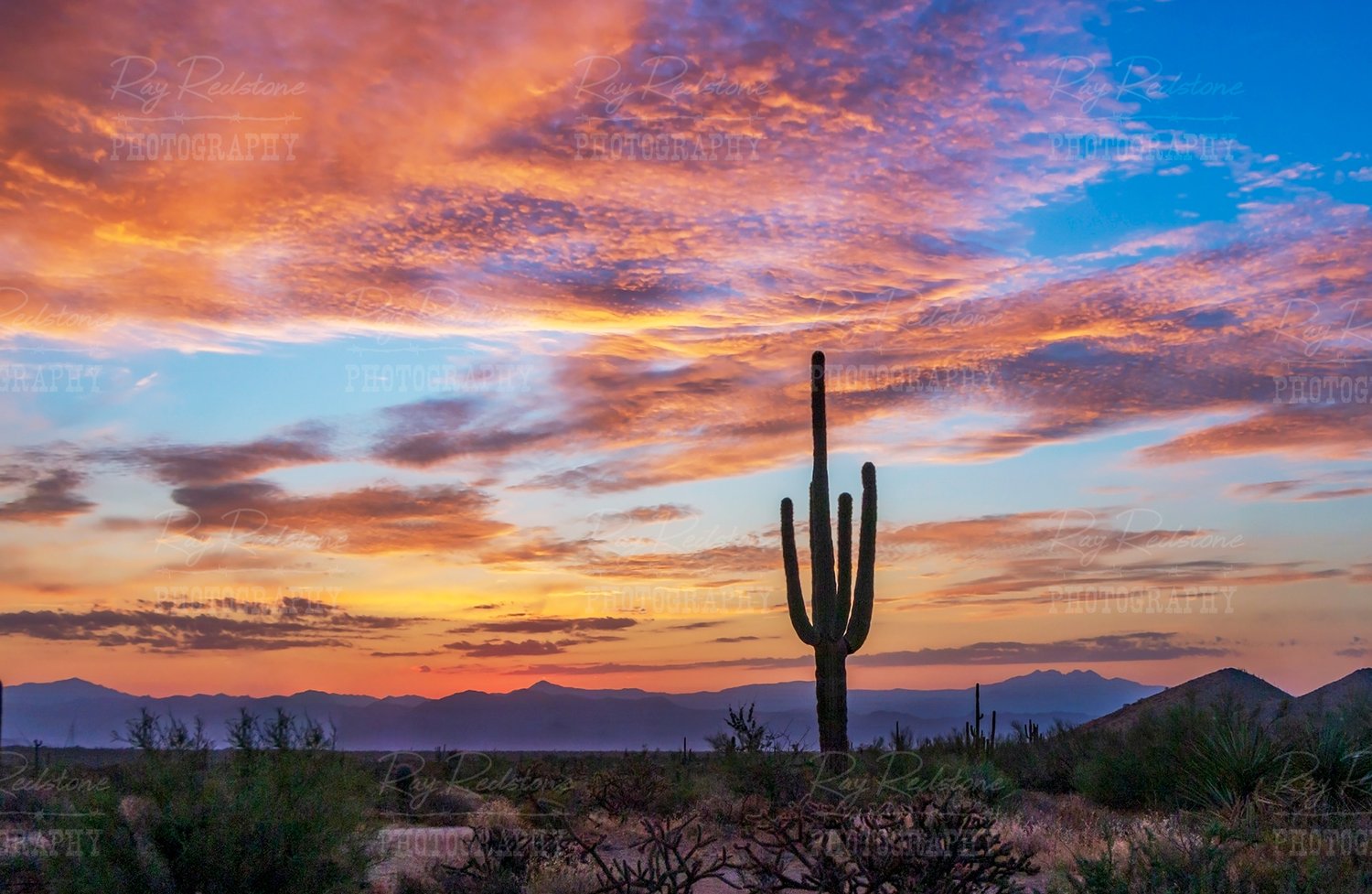This photograph captures an expansive desert landscape reminiscent of Arizona, though it might also be from Nevada or Utah. The sky is painted in stunning sunset hues, featuring vibrant oranges, pinks, yellows, and purples, with patches of blue still visible. The horizon is predominantly orange, and distant mountain silhouettes can be seen far away, with closer rugged peaks adding depth to the scene. Dominating the foreground is a tall saguaro cactus just to the right of center, accompanied by various desert plants, including scrub brush, smaller cacti, and possibly small Joshua trees. The sandy terrain suggests a faint road, bordered by scattered vegetation leading towards the mountains. Throughout the image, faint watermarks reading "ray redstone photography" subtly mark the piece, enhancing its authenticity while not detracting from the breathtaking beauty of the desert at sunset.